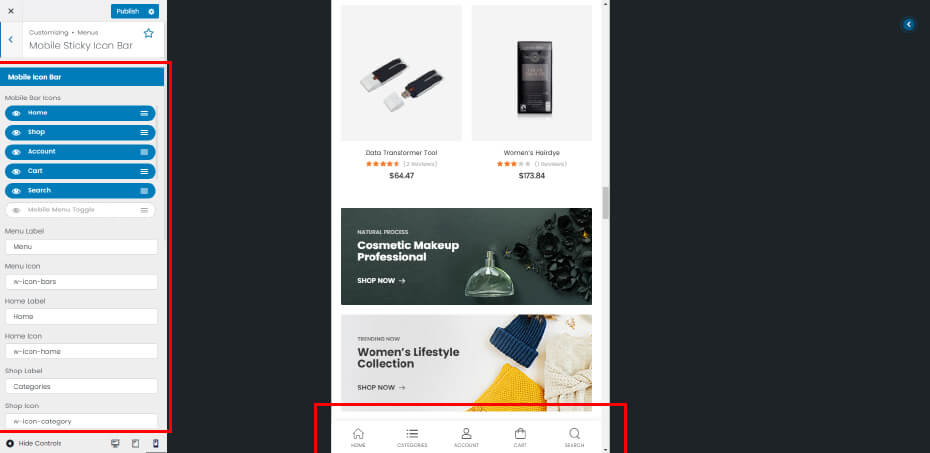The image depicts a detailed screenshot of a web page from Cosmic Makeup Professional. Dominating the center is a pop-up message in grey text urging visitors to "Shop Now." 

The web page's layout is segmented with distinctive features. The left side features a grey and white background adorned with horizontal blue bars, stretching from the top and continuing down the side. This gray and white section, accented by blue bars, is neatly outlined in red.

Adjacent to this, a substantial black column extends from the top edge of the page to the bottom. Within the central part of the page, various advertisements and purchasable items are displayed. At the top, two products are prominently showcased in black and white images, complete with price tags.

Beneath the pop-up, there is a "Women's Lifestyle Collection" section featuring a blue hat, a yellow scarf, and an off-white sweater. Further down, another red-outlined box marks the home area, containing multiple icons and a subscription sign-up section.

Approximately two-thirds of the page to the right is enveloped by a solid black screen, adding a dramatic contrast to the rest of the page's design.